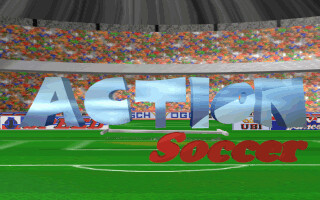A vibrant 3D-rendered title screen of a video game set in a bustling soccer stadium. The stadium's stands are packed with a diverse, colorful crowd, creating a lively atmosphere. The field itself is a lush dark green with clearly marked white lines, accurately depicting a soccer pitch. Dominating the scene, the title "ACTION SOCCER" is prominently displayed: the word "ACTION" is written in large, cartoony letters that transition from dark blue to light blue hues with a hint of a sky or water texture, while "SOCCER" is rendered in a bold red gradient. Above the stands, there is a domed roof with black, dark gray, and light gray stripes, adding depth to the scene. The overall composition suggests an engaging and dynamic sporting event, capturing the excitement of the game.